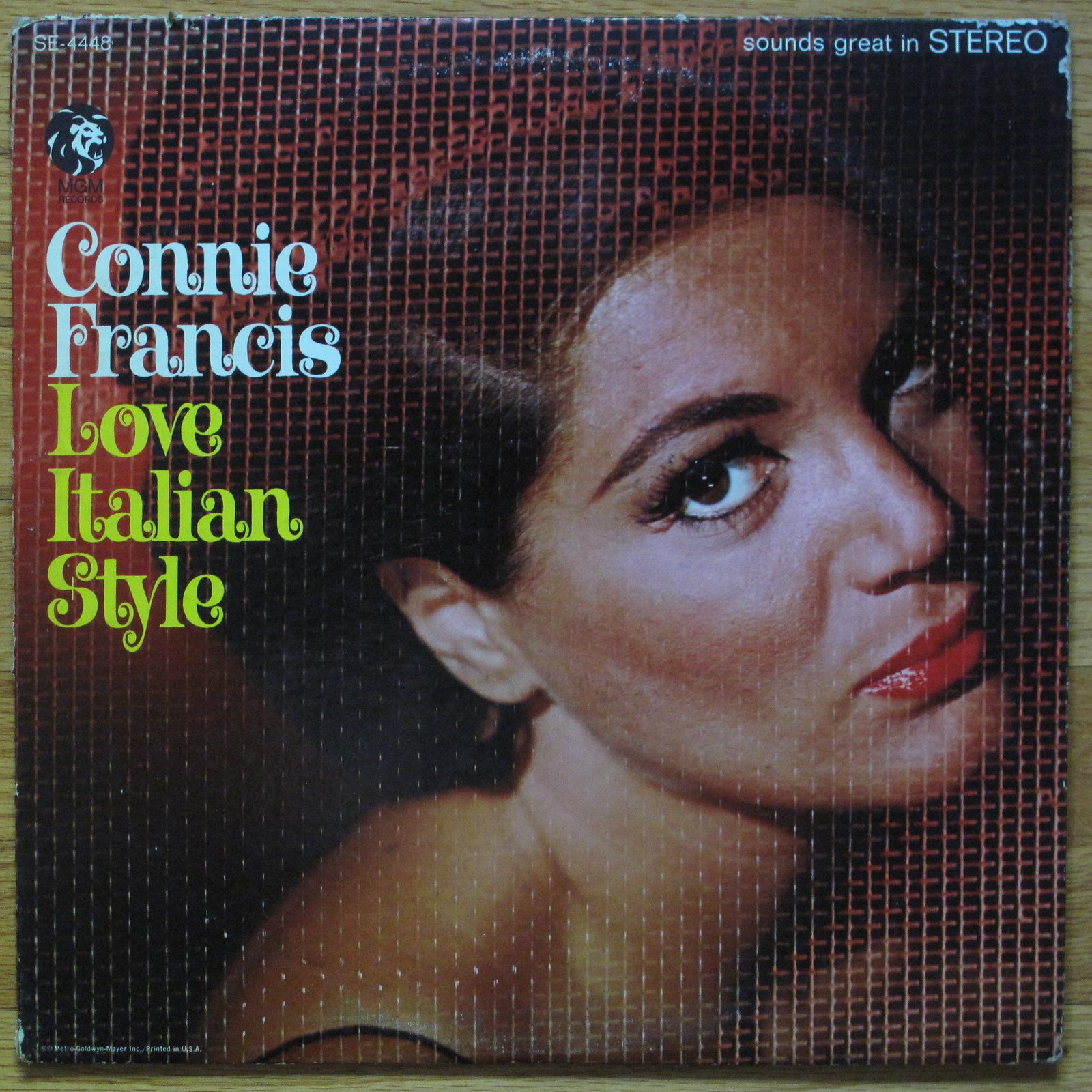This poster or album cover features a striking profile photograph of a woman, who turns to look back at the camera. She has bold red lipstick, brown eyes, and dark brown hair. She appears to be either shirtless or wearing a strap over her right shoulder, which is brown in color. The background is a pattern of red, black, and what seems to be a checkerboard or chain-link fence texture, giving it a distinct graphical feel. 

Prominent text includes "Connie Francis" in white cursive letters, followed by "Love Italian Style" in yellow text beneath it. This text is positioned over a backdrop that appears to be light brown wood. The top right corner of the cover features the words "Sounds Great in Stereo" in white letters, with "Stereo" in all caps. The catalog number "SE4448" is written in the top left corner. Additionally, the album cover includes a logo of MGM Records on the left side towards the top, and a white lion head just below it. The overall design and detailed elements contribute to a vintage and stylized presentation, akin to an album from the 1940s.